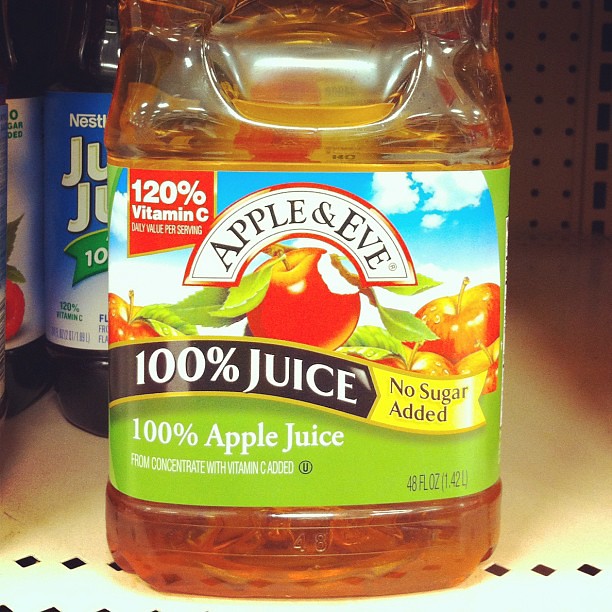A meticulously organized white metal shelf prominently displays juice bottles. On the left, two bottles of 'Juicy Juice' stand out with their distinctive blue labels, showcasing a vibrant purple-colored juice. The labels are both eye-catching and uniform, creating a visual harmony. To the right, an 'Apple & Eve 100% Apple Juice' container is slightly moved forward, almost at the edge of the shelf, subtly overlapping the 'Juicy Juice' bottles. The 'Apple & Eve' juice bottle, with a label specifying "No Sugar Added" and a content volume of 48 fluid ounces (fl oz), is highlighted. The label also mentions that the juice is made "From Concentrate with Vitamin C Added," and it features a certification symbol—a black outlined circle with a black 'U' inside it—indicating it meets certain standards. The right side of the shelf appears spacious and uncluttered, emphasizing the careful placement and selection of the featured juice bottles.